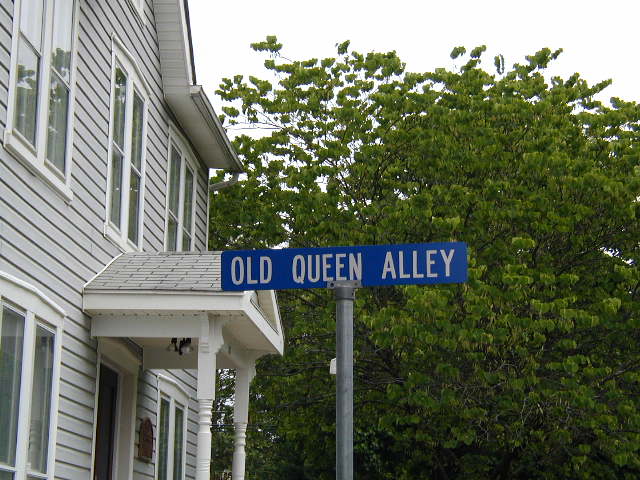A spacious blue house with two levels stands prominently, adorned with contrasting white trims. A towering tree with lush green leaves stretches almost to the height of the house. The sky is shrouded in a light fog, casting an off-white hue over the scene. In the foreground, a cylindrical metal pole supports a blue sign with white lettering that reads "Old Queen Alley." The house features two porch lights flanking the entrance door, where another decorative sun motif is displayed.